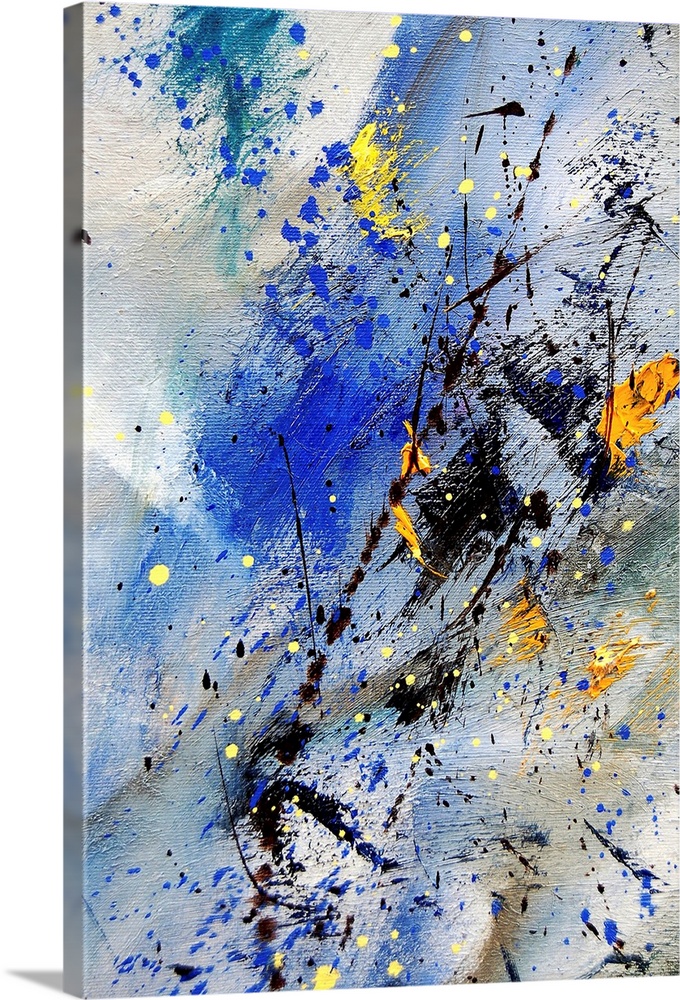This modern abstract art piece, displayed on a canvas, bursts with vivid colors and captivating textures. The horizontally rectangular, nearly square painting showcases a dynamic blend of brush strokes and paint splatters. The mostly white background serves as a canvas for the chaotic, yet intriguing, application of colors, including various shades of blue, black, gray, mustard yellow, lemon yellow, teal green, orange, and tan. 

On closer inspection, the upper left-hand corner features blue spatters running down the center, while black paint speckles streak vertically from bottom to top, creating a sense of movement. The texture varies across the painting, with some areas showing thick, layered paint, giving it a three-dimensional quality. Interestingly, if you tilt your head to the right, the disorganized paint splatters might resemble a human face, with a wide curve at the bottom possibly representing lips, a diagonal line suggesting a cheek, a dark diamond shape resembling an eye, and a triangular black swipe hinting at a nose. Despite its abstract nature, this complex interplay of colors and textures invites interpretation and engages the viewer's imagination.